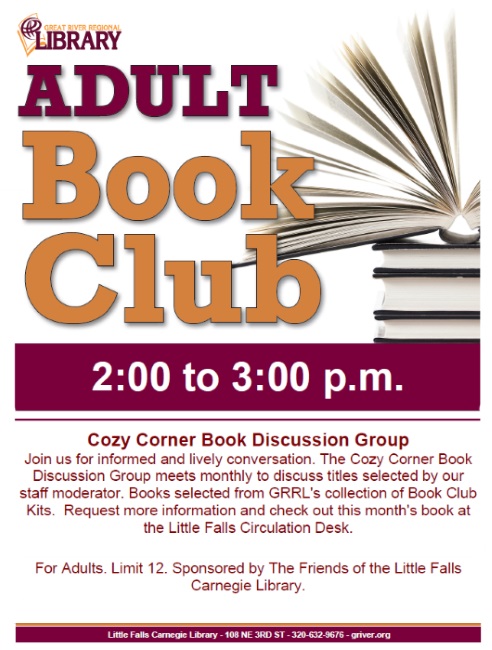Great Rivers Regional Library Poster

This library poster features maroon and mustard yellow lettering on a white background with deep red and orange highlights. The poster announces the "Adult Book Club," which meets from 2:00 to 3:00 p.m., and introduces the "Cozy Corner Book Discussion Group." The group gathers monthly for informed and lively conversations, moderated by the library staff. The chosen titles come from the GRRL's collection of book club kits. Attendees can request more information and check out the month's book at the Little Falls Circulation Desk. Participation is limited to 12 adults and is sponsored by the Friends of the Little Falls Carnegie Library.

On the right side of the poster, there is an image of a stack of three closed books with a fourth book fanned open on top. The detailed banner under the club information includes the address: Little Falls Carnegie Library, 108 NE 3rd Street, phone number 320-632-9676, and website GRiver.org. Note: There is some smaller, unreadable text on a banner at the bottom of the poster.